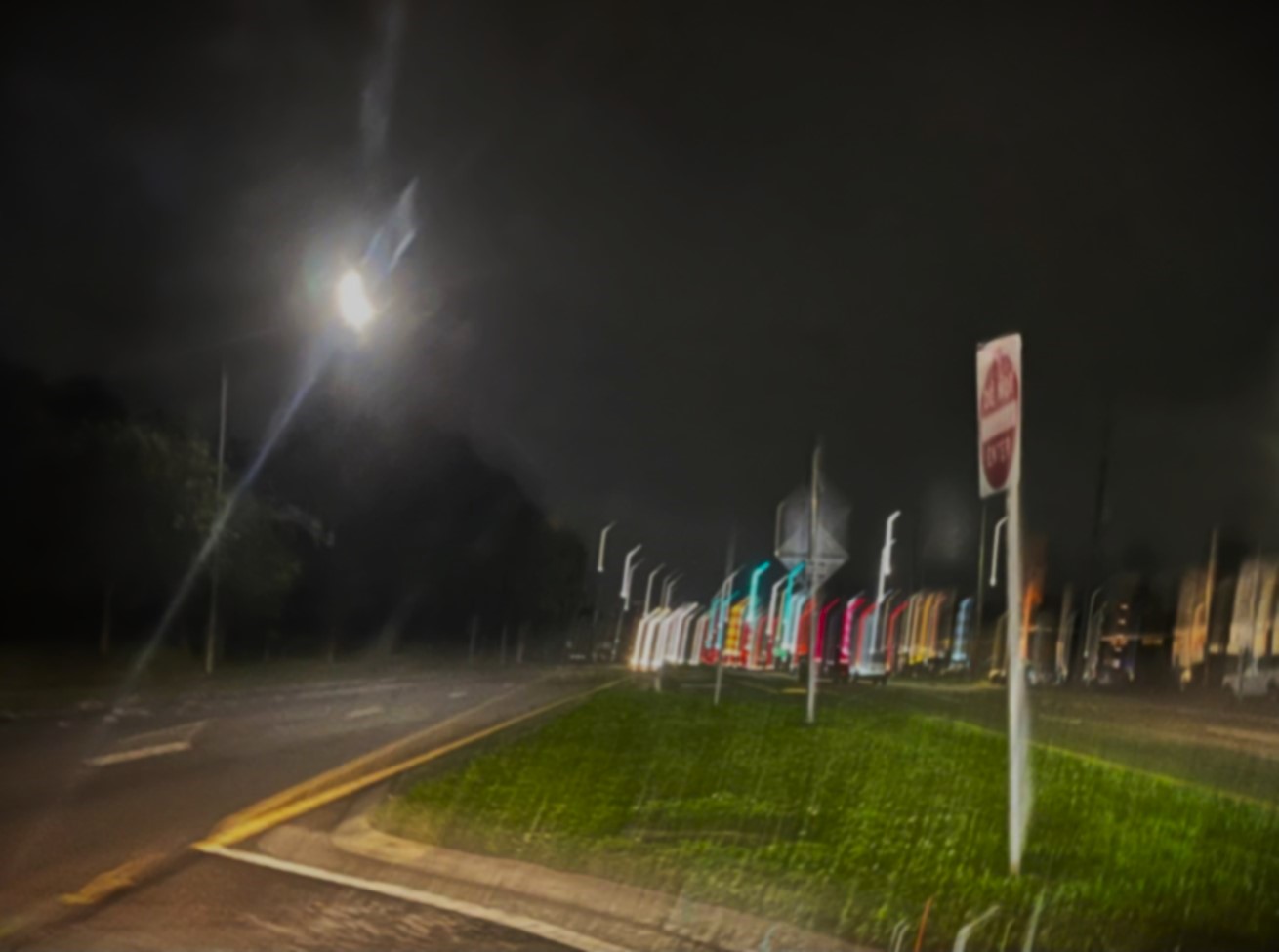This nighttime outdoor photo captures a blurred street scene, likely because of low light and possible rain. The roadway stretches horizontally from the bottom left to the upper section of the image. On the left side of the road, there is a bright streetlamp illuminating the scene. Adjacent to the roadway on the right is a plot of grass with a curved edge, flanked by roads on both sides. A prominently visible "Do Not Enter" sign with white capital letters on a red circle stands on a metal pole in this grassy area. Various flares and light streaks of white, blue, yellow, red, and orange colors appear throughout the image, contributing to its hazy and indistinct appearance. In the background, there are blurred buildings or structures featuring red, white, and yellow lights, adding to the night-time ambiance.